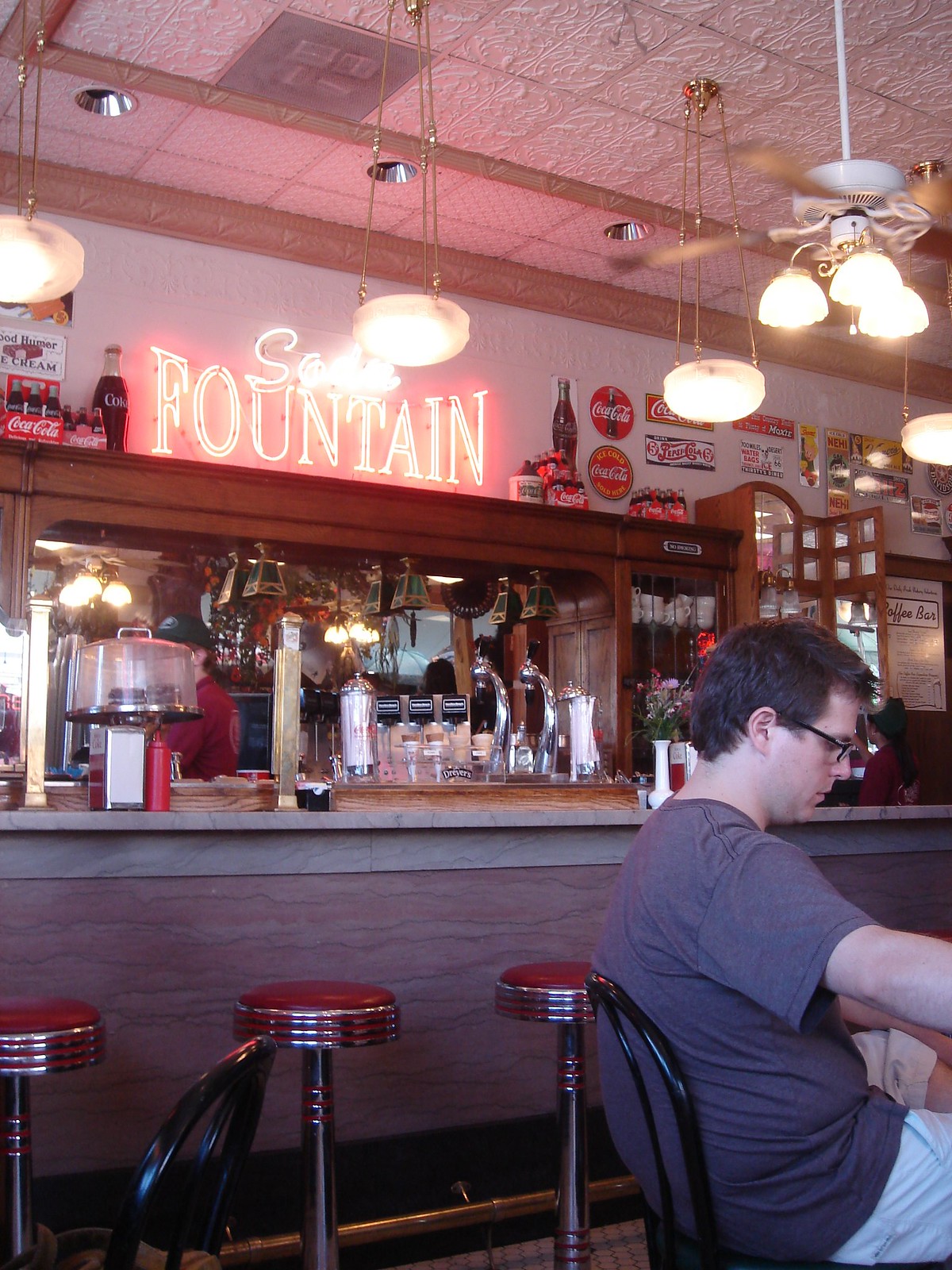The image captures the inside of a nostalgic bar, a drinking establishment adorned with Coca-Cola memorabilia. Central to the scene is the marble bar, lit warmly by a mix of hanging light fixtures on gold chains, inlaid lighting, and ceiling panel lights. Above the bar, a prominent bright red neon sign reading "Soda Fountain" takes its place, surrounded by an array of Coca-Cola advertisements, bottles, and light wood cabinets.

The bar itself is furnished with retro bar stools featuring steel posts, red vinyl tops, and chrome accents. On the bar, a bottle of ketchup, some napkins, and a stand displaying cakes create a casual, inviting atmosphere. To the distance, a coffee bar is noticeable on the wall. Adding a touch of charm, a bunch of flowers complements the scene.

In the bottom right corner, a patron is depicted sitting in a black chair, wearing glasses and sporting short brown hair. He has on a brown t-shirt and white pants, attentively looking down at the table, possibly reading a menu. The overall environment, enhanced by a pinkish hue from the lights, reflects a cozy, old-fashioned ambiance.